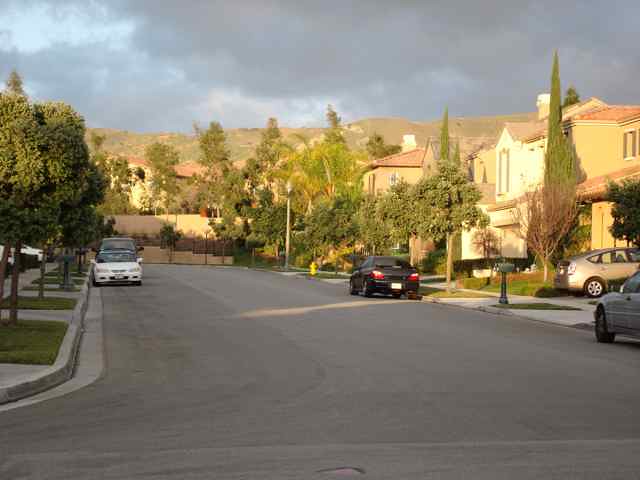This detailed image captures a typical suburban street likely in Arizona or New Mexico. The scene portrays a meticulously maintained residential area with single-family homes, some of which are two-story with multiple rooms. The houses are standard creamish-brownish with darker brown tannish roofs, resembling terracotta structures. Lining the road are trees planted between driveways, enhancing the suburban feel. Several cars are parked along the side of the road and in driveways. Despite a predominantly cloudy sky that casts a golden hue over the neighborhood, sunbeams intermittently break through, reflecting off the sides of houses and illuminating spots on the ground. The backdrop features a scrubby hill or a big dirt mound, devoid of greenery. This careful blend of natural and built elements creates a serene yet arid suburban environment characteristic of the American Southwest.